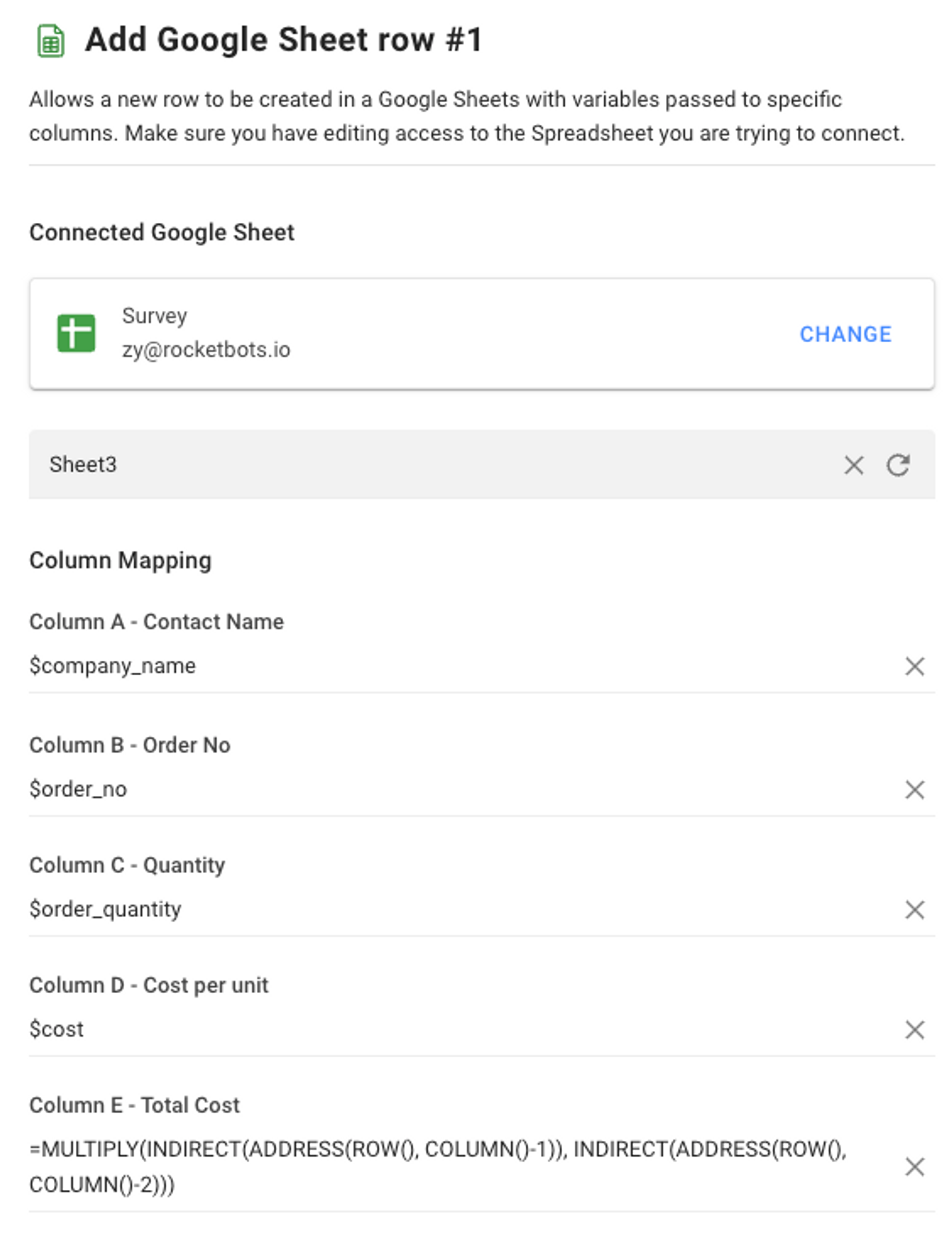This screenshot, taken from within the Google Sheets app, showcases a detailed configuration screen. The page features a simple white background with black text. At the top left corner, there is a small icon that represents a spreadsheet page. Adjacent to it on the left, "Add Google Sheet" is mentioned, followed by the heading of row number one in bold black text. Directly below, there is a paragraph discussing variables.

Further down, a section labeled "Connected Google Sheet" is enclosed within a gray-outlined box. Inside this box, on the left, there is a dark green icon with a white off-sided cross. To the right of this icon, the text displays "Survey" alongside an email address: xi@rocketbots.io. On the far right of this section, the word "Change" appears in blue text.

Below this, a horizontal gray banner states "Sheet number three" on the left, accompanied by an "X" and a reload icon on the far right. The subsequent section, titled "Column Mapping" in bold black text, maps out various columns from the sheet.

- Column A is labeled "Contact Name" with a reference to "$company_name" on the left and a black arrow pointing to the right.
- Column B is labeled "Order Number" with a reference to "$order_number" and an "X" on the right.
- Column C, marked as "Quantity," references "$order_quantity."
- Column D, titled "Cost per Unit," references "$cost."
- Column E, labeled "Total Cost," contains a formula: =MULTIPLY(INDIRECT(ADDRESS(ROW(), COLUMN())), INDIRECT(ADDRESS(ROW(), COLUMN()))). 

Each row in this section ends with an "X" on the right side, indicating options for deletion or modification. This detailed screenshot provides a clear view of the data structure and operations set up within the Google Sheet.